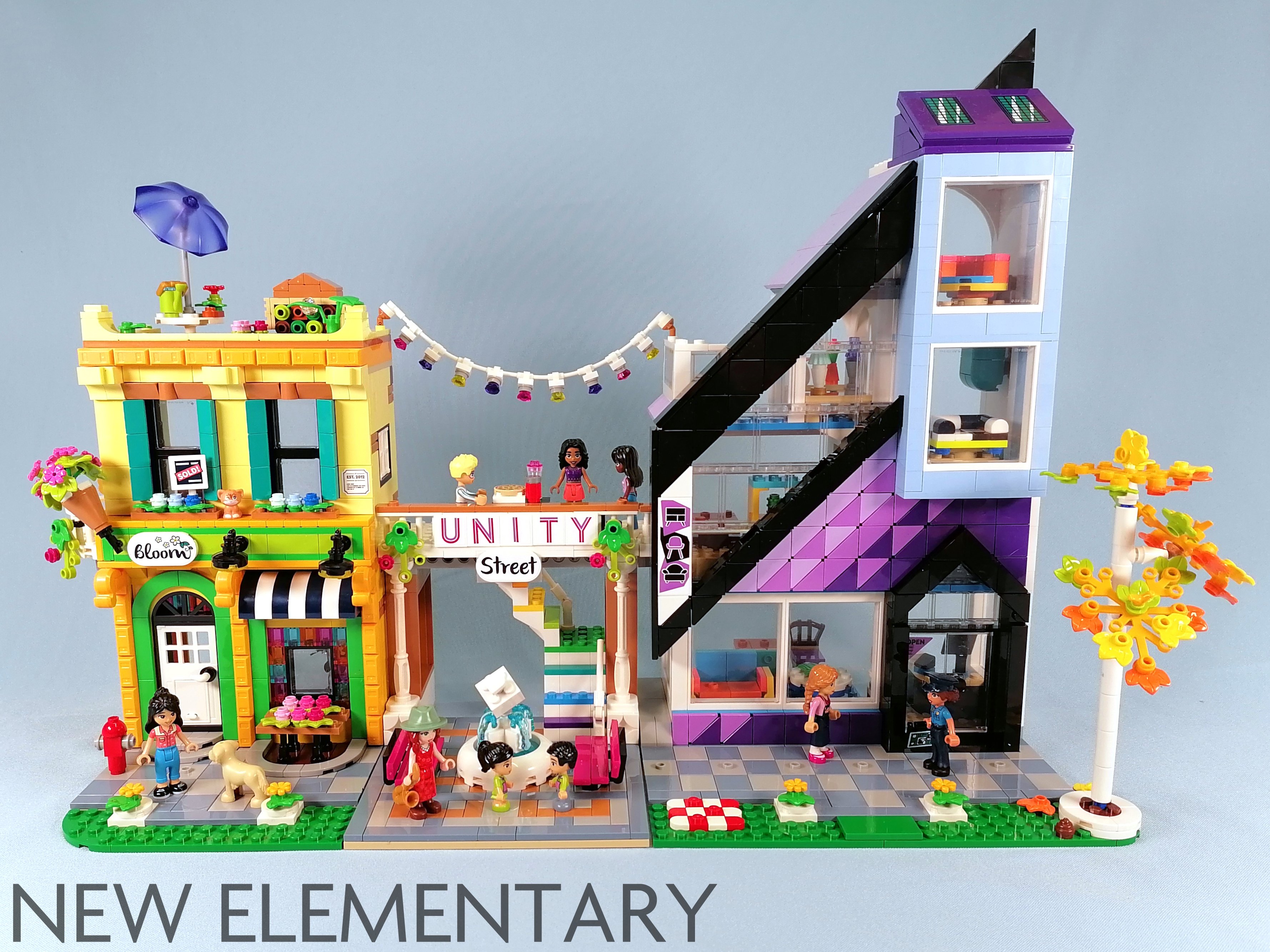The image depicts a detailed Lego playset resembling a vibrant community street scene. On the left-hand side, there's a two-story yellow building with a green bottom and a yellow top. The front half of this building features a white door and a woman dressed in blue pants and a red striped shirt standing with her dog near a fire hydrant. The center of the scene showcases an archway with a white background and red lining that reads "Unity," surrounded by people who appear to be eating, celebrating, and engaging with each other near a fountain.

To the right, a modern, taller building rises with a sleek, angled black top and a glass facade adorned with light purple and pink tiles. This structure, which appears to be a multi-level apartment or house, has a chair visible and is accompanied by figures of a female and a police officer in front. The scene includes various elements such as a tree with orange leaves, a florist booth labeled "Bloom" with an umbrella and purple stairs, and green Lego pieces representing grass. The entire setup is placed against a baby blue background with bold grey text at the bottom corner that reads "New Elementary." The figures within the playset are varied, suggesting a lively, communal atmosphere.